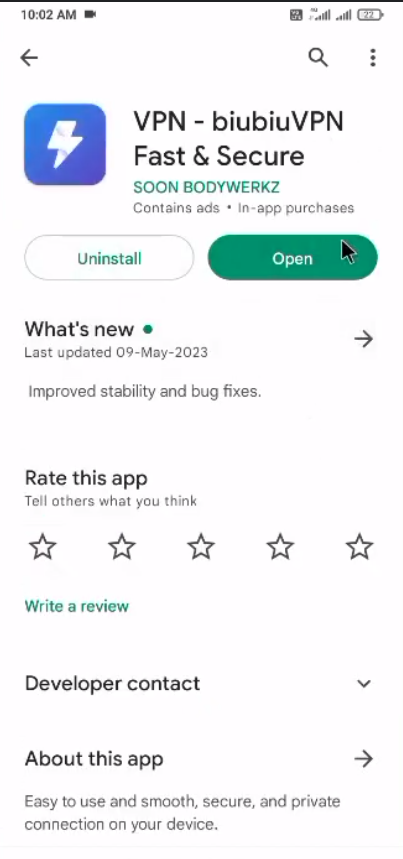This screenshot depicts the Google Play Store page for the app "BIUBIU VPN - Fast & Secure," developed by Soon Body Works. The page features options to "Uninstall" or "Open" the app, indicating it is already installed on the user's device. The app's listing notes that it "Contains Ads" and offers "In-app Purchases." The app was recently updated on May 9th, 2023, with improvements in stability and various bug fixes.

The "about this app" section and a "developer contact" option are accessible, giving users further information about the app and a way to reach out to the developers. The page maintains a light mode display, with a white background and most of the text in black. The "Open" button stands out in green with white text, while hyperlinks are displayed in green for easy identification. 

The app's logo features a simple blue square with a white lightning bolt. Users are invited to rate the app, with the review option offering a star rating system out of five.